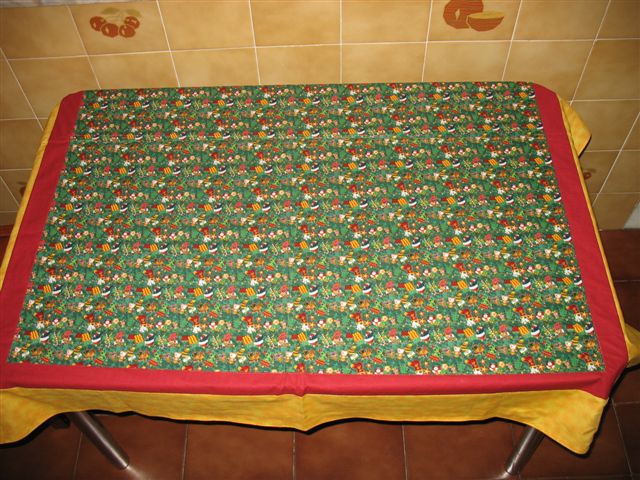In the image, a small rectangular table is situated in a kitchen, its surface beautifully adorned with a meticulously designed tablecloth. The tablecloth fits the table perfectly and features a striking red border that frames intricate multi-colored designs in the center. Predominantly, the middle of the tablecloth showcases varied hues of green, supplemented by patterns in yellow, red, black, white, and some delicate motifs in mustard yellow and lighter orange – possibly floral. The bottom edge of the tablecloth is accentuated with a yellow or gold trim. 

The table itself has slender metal legs, hinting that it might be folded. In the background, the kitchen walls are adorned with light brown or tan tiles, interspersed with occasional tiles that carry charming fruit illustrations, like olives and a fruit bowl, adding to the room's rustic charm. The flooring consists of bronze-colored tiles enhancing the warm aesthetic of the space. The table dominates the foreground, covering a substantial portion of the image, emphasizing its intricate tablecloth and the harmonious kitchen setting around it.